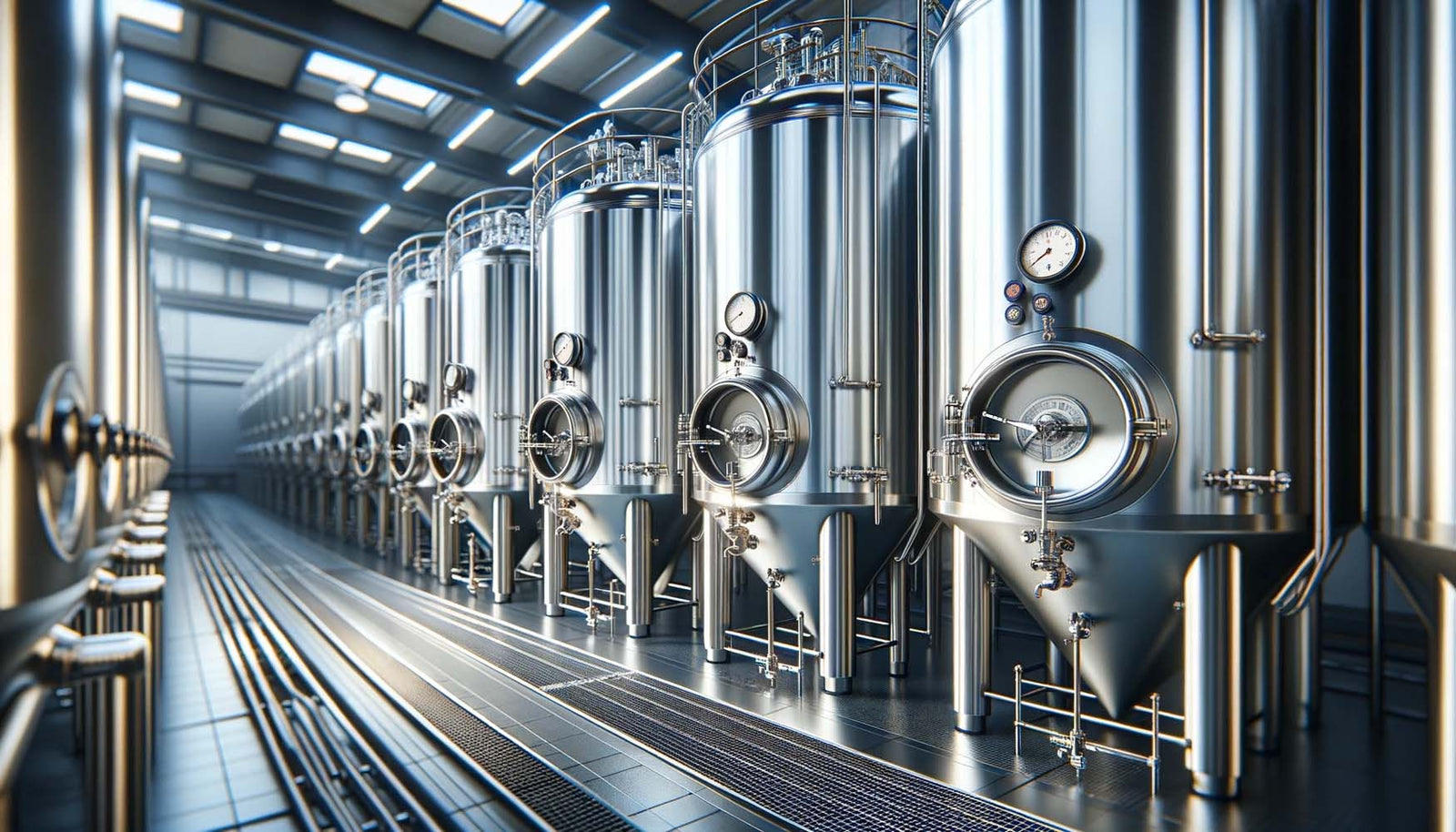This image captures a highly industrial brewery interior featuring a long, symmetrical corridor lined with large, stainless steel fermenting vats. The vats are cylindrical, with reflective surfaces and are prominently equipped with dials, pressure gauges, and nozzles. Each vat tapers into a conical bottom and is supported by metallic pedestals. The vats are organized in parallel rows, stretching down the length of the room on both sides, creating a scene that almost seems endless and uniformly metallic. 

Above, recessed and fluorescent lights illuminate the space, with additional natural light streaming in through large, high windows, accentuating the brightness of the steel. The room itself has walls and floors that complement the shiny metal theme, enhancing the industrial atmosphere. The floor features grates running centrally beneath the vats, likely for drainage or piping. Despite its realistic appearance, the scene exudes a synthetic, almost computer-generated quality due to its impeccable organization and uniformity.